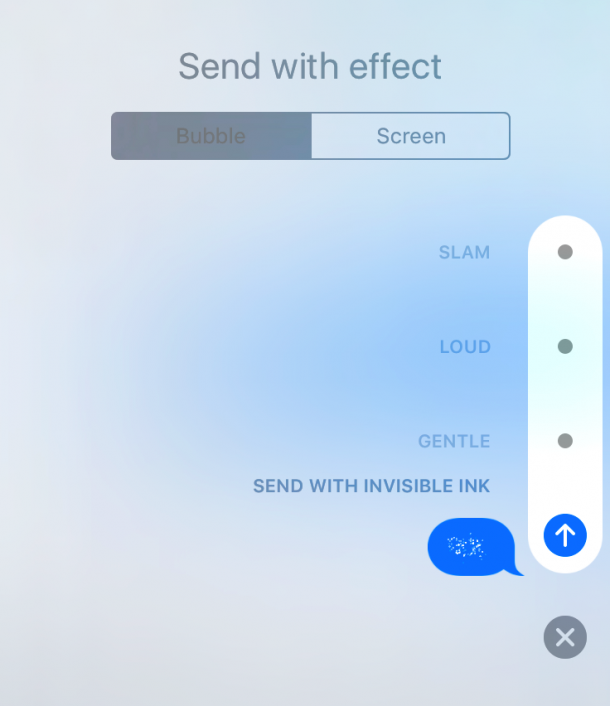In this image, the background displays a stunning tapestry of clouds in shades of white, blue, and hints of pink. The lower third of the image is predominantly pink, transitioning into mostly blue toward the top right corner. At the center, gray text reads "Send with effect," positioned above a rectangular box presenting two options: "Bubble" on the left, which is darkened and highlighted, and "Screen" on the right. On the right side of the image, a white, oblong, vertical bar is visible. To its left, in light blue text and arranged vertically from the top, the options include "Slam" with a gray dot beside it, "Loud" with a gray dot to the right, "Gentle" with a gray dot to the right, and beneath these, "Send with invisible ink."